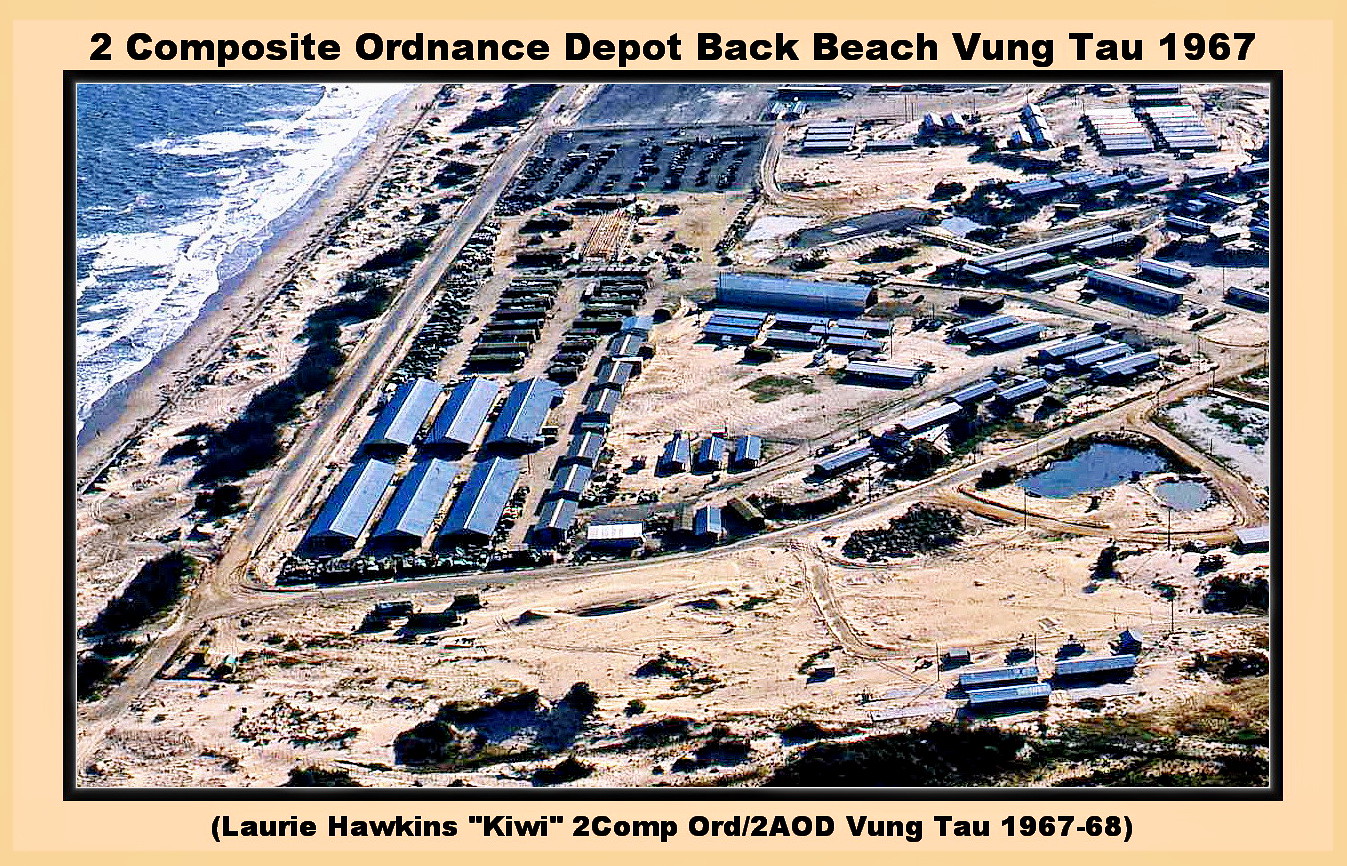This detailed image is an outdoor, daylight, aerial color photograph of a military base situated on a beach named Vung Tau, specifically labeled "Two Composite Ordnance Depot, Back Beach, Vung Tau, 1967" along the top border. Additional text at the bottom reads "Lori Hawkins Kiwi 2 Comp Ord/2 AOD Vung Tau 1967-68." The photograph is bordered first by black, and then by a thicker, off-white, yellowish border.

In the photograph, you can see the ocean to the right, with surf and waves breaking upon a sandy beach area. The land itself is predominantly light brown, appearing as sand or bare dirt, with little to no grass. A network of dirt roads and paths crisscrosses the landscape, leading to numerous long, low, peaked-roof buildings which appear to be warehouses or similar structures rather than houses. 

A large black parking lot is visible, crowded with various vehicles like trailers and trucks. Additionally, there are several small lakes or drainage ditches filled with water, particularly notable is one surrounded by a perimeter road. Sparse dark green vegetation is present in the bottom right and along a road by the beach. The photograph presents a scene characterized by an expanse of flat, open ground with scattered military infrastructure and minimal greenery, emphasizing its functional and utilitarian nature.